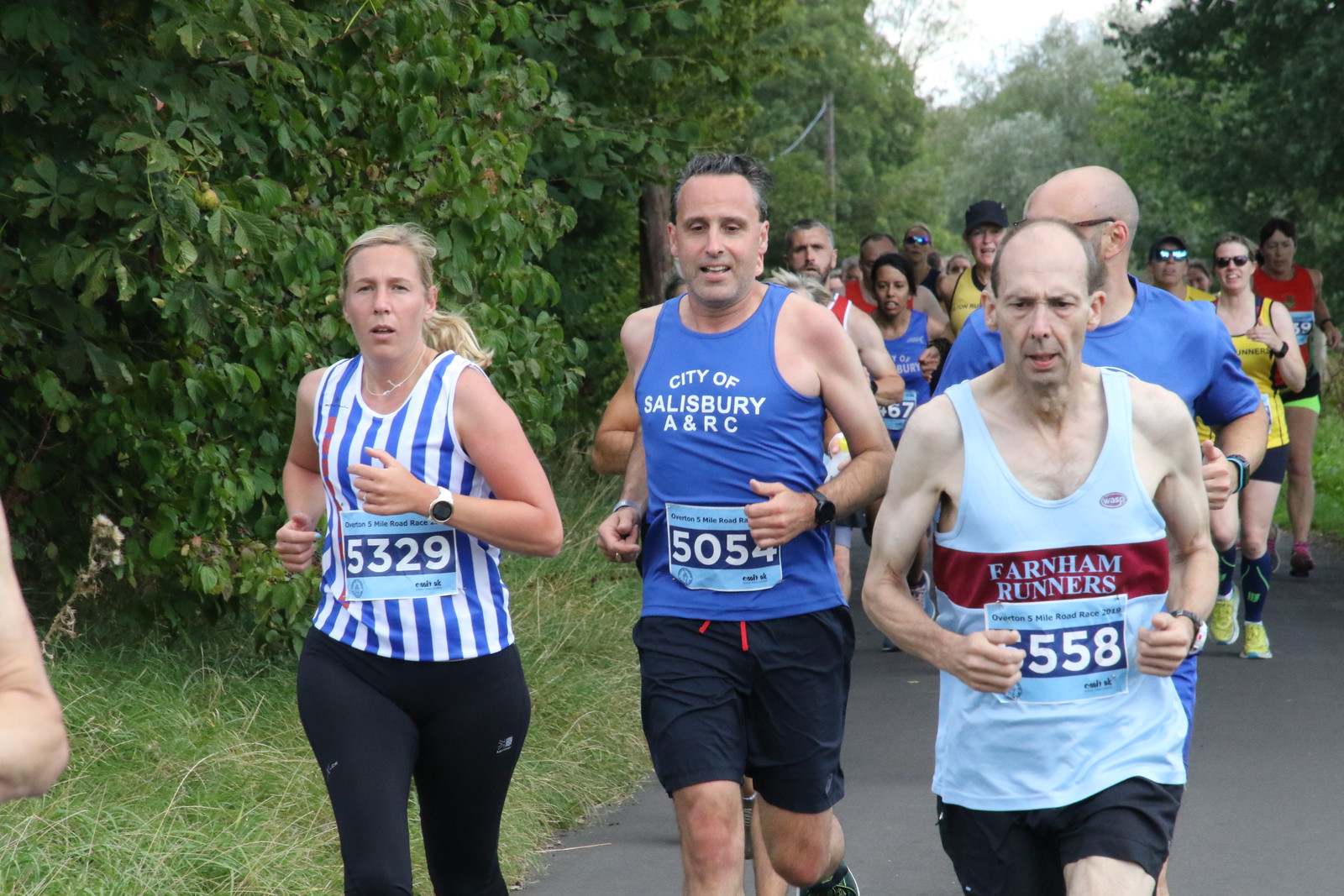This is an outdoor photograph capturing a segment of a marathon on a somewhat overcast day. The image frames a group of runners, prominently featuring three individuals in the foreground. The closest to the camera is an older, bald man with graying hair at his temples, wearing a loose-fitted light blue tank top that reads "Farnham Runners" and black shorts. His runner's number, mostly obscured by his hand, reads 558. To his left, another older gentleman with gray and black hair is seen in a blue tank top with the inscription "City of Salisbury A&RC" and the runner's number 5054 prominently displayed. Further to the left is a woman with long blonde hair pulled into a ponytail. She is wearing a blue and white vertical striped tank top and black running tights, with the number 5329 visible on her front. The runners are moving along a smooth, gray paved path flanked by green grass and tall trees, providing a scenic backdrop. In the background, various runners of different ages and ethnicities can be seen, each adorned in athletic wear with their race numbers attached, participating in this energetic event.